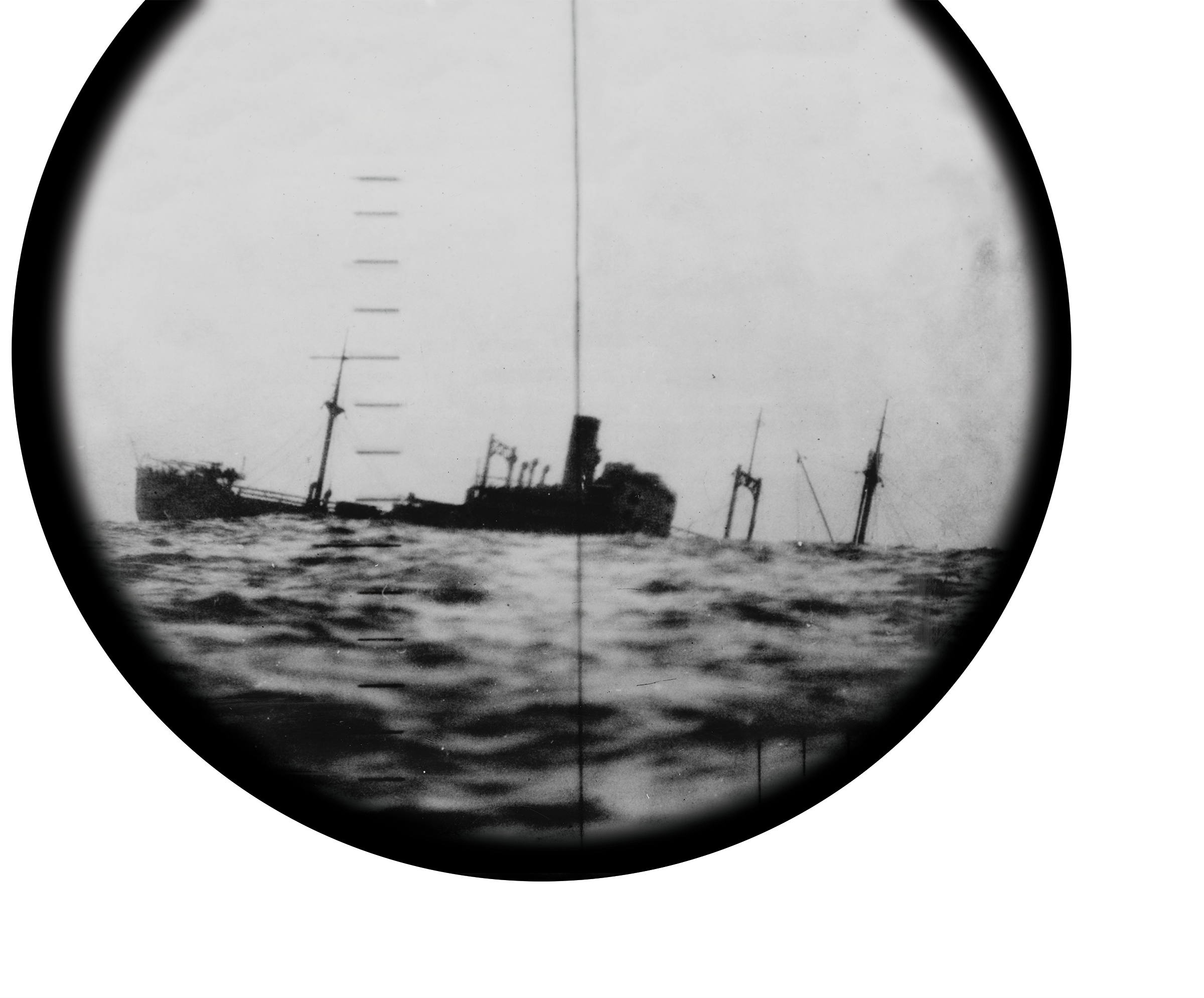The image is an old, black and white photograph, viewed through a circular frame reminiscent of a periscope or submarine viewport, with the top portion of the circle obscured by a black frame. The photo is slightly blurry, with increased blurriness towards the edges, and lacks strong contrast, lending it a very vintage appearance. The scene depicts a vessel on wavy waters, appearing to be in the process of sinking. The front part of the ship is still visible above the water, tilted at an angle, while the middle section, including what appear to be towers or the upper deck, is gradually vanishing below the waterline. The sky above the scene is a blank, featureless white, further emphasizing the old, perhaps historic nature of the photograph.